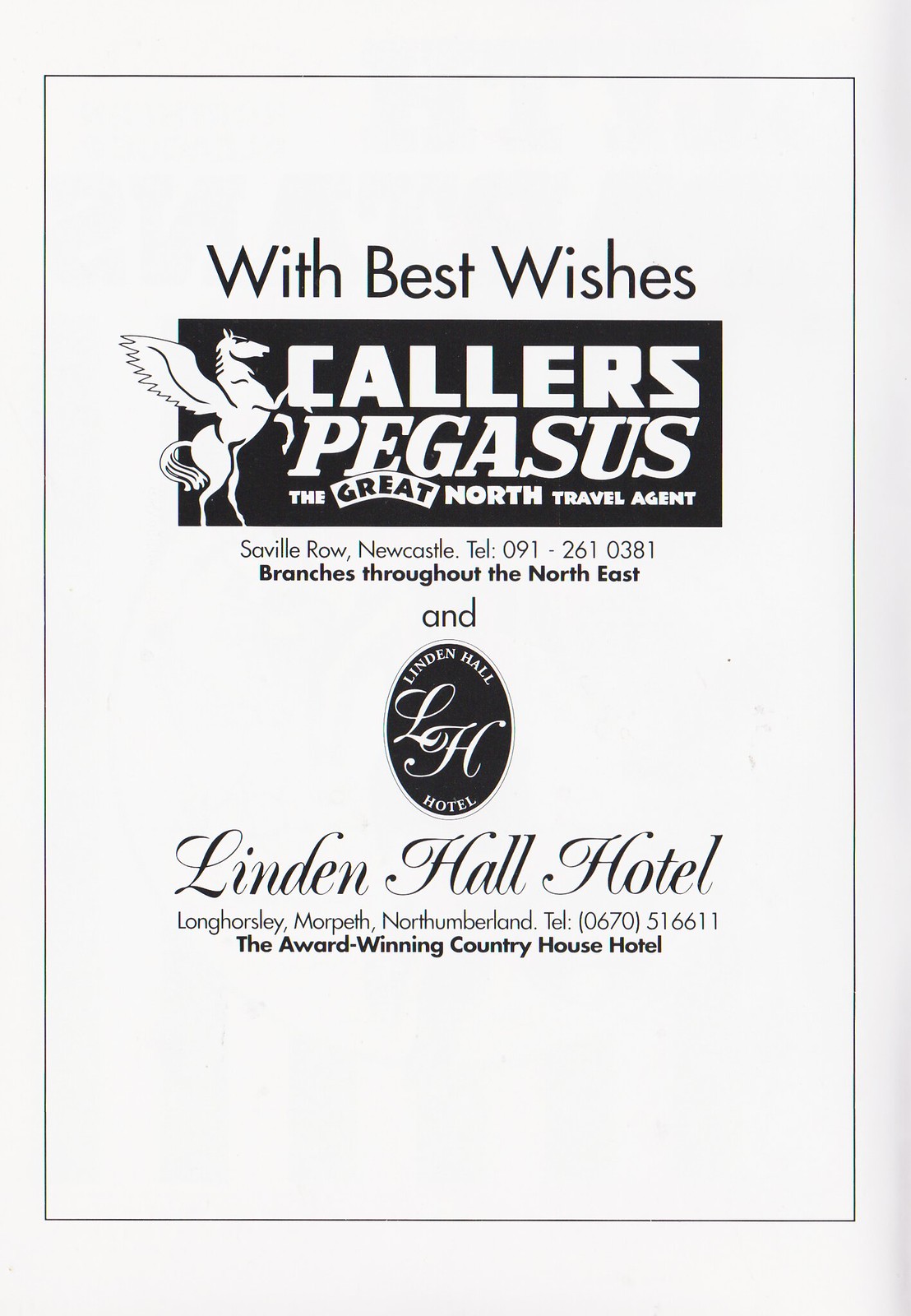A business flyer with a clean white background featuring black text and imagery. At the top, in black capital letters, it reads "With Best Wishes." Below that is a black rectangle with the words "Collar's Pegasus" in large white capital letters, with "Pegasus" in italics. To the left of this text, there is an image of a Pegasus horse rearing on its hind legs. Underneath the rectangle, in smaller black letters, it states: "The Great North Travel Agent." 

Further down, the flyer provides the contact details: "Savile Row/Newcastle, Tel: 091-261-0381," and mentions that there are branches throughout the Northeast. Below this, there is a black oval image with the abbreviation "LH" in white, and in cursive, the text "Linden Hall Hotel," with the hotel's address and phone number listed underneath.

Overall, the flyer presents a polished, monochromatic advertisement blending textual details and illustrative elements for Collar's Pegasus and Linden Hall Hotel.